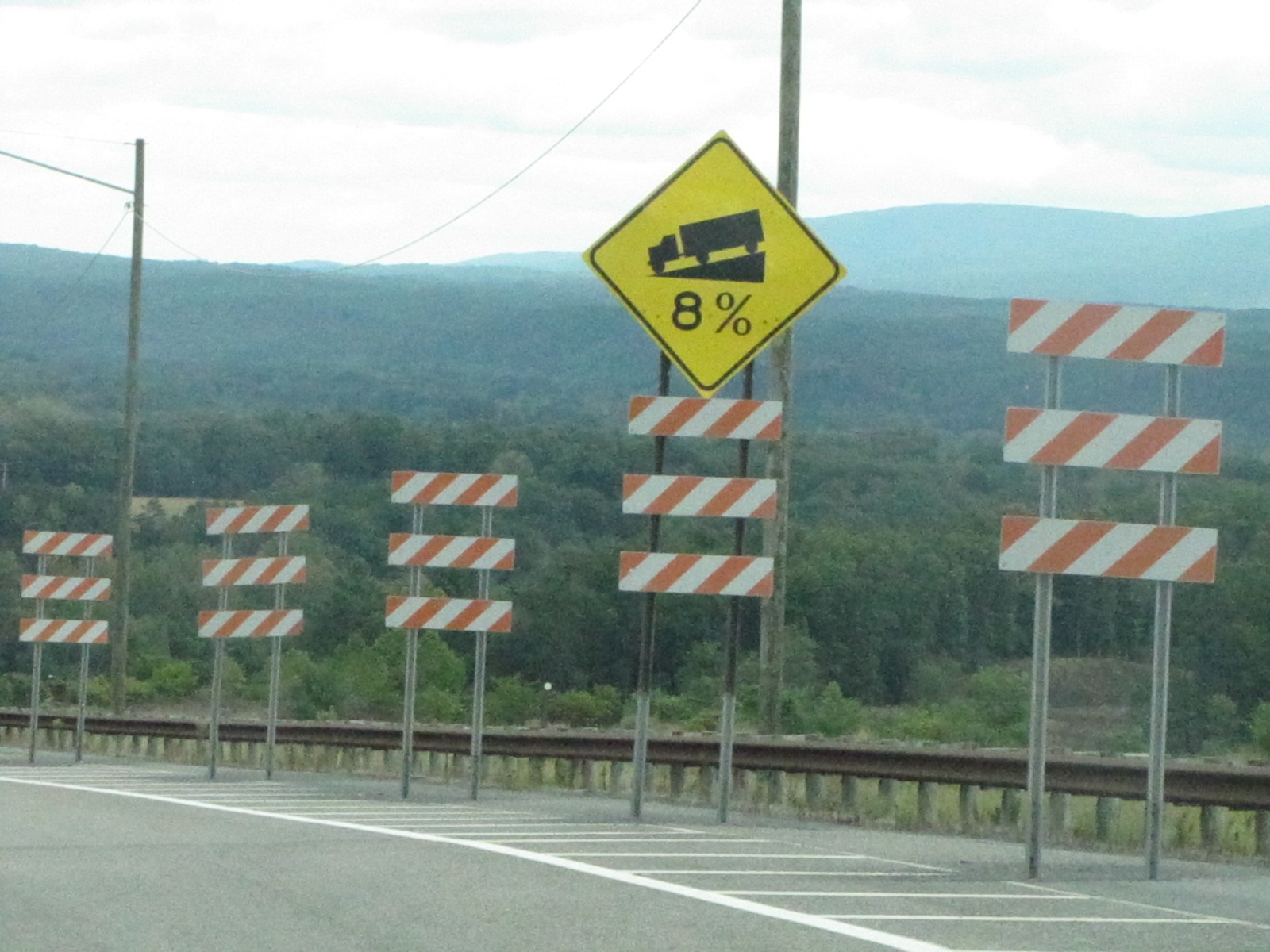A square-shaped outdoor photograph captures a serene landscape under a predominantly cloudy sky, creating a soft white hue above. In the background, majestic mountains rise, complemented by a sprawling field of vibrant green trees. The foreground presents a gray road marked with white lines, flanked on the side by five distinctive signs, adorned in white and orange. Among them, a prominent diamond-shaped yellow sign with bold black markings warns of a truck descending a steep incline, adding a touch of dynamism to the tranquil scene.